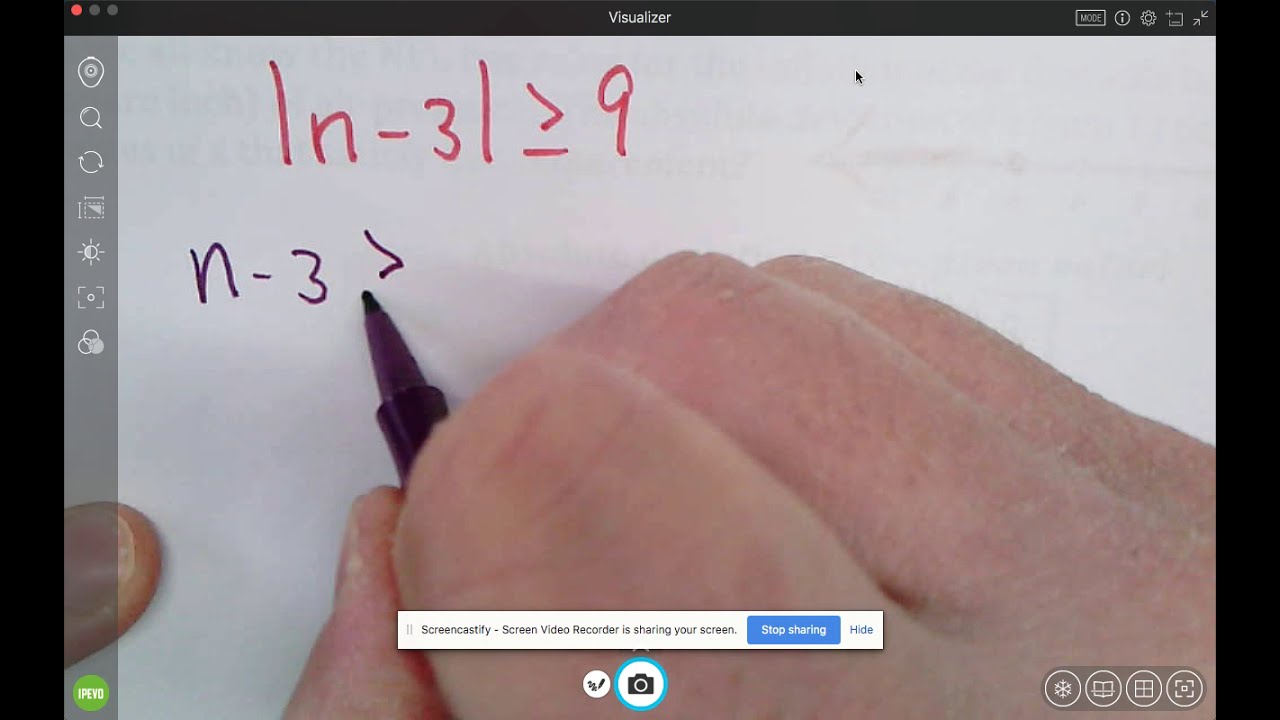The image displays a detailed screenshot of an online math lesson, captured in landscape orientation. The focal point is a man's right hand holding a black pen, actively writing a math equation on a whiteboard. The board shows two lines of handwritten text: the first equation, "absolute n minus three is greater than equal to nine," is written in red ink across the upper left-hand corner, while the second line of text is in black ink, being written out beneath it.

In addition to the whiteboard content, the screenshot includes several interface elements indicative of an online teaching session, likely conducted via Skype or a similar platform. At the top center, a black bar displays the word "Visualizer" in white text. The upper left corner features three small dots with the leftmost dot filled in red, suggesting that recording is in progress. On the top right, there are several small, unreadable icons and a symbol resembling an eye in a circle.

Along the left side of the screen, a vertical gray navigation panel includes options for adjusting brightness, refreshing the screen, and zooming in. At the bottom, a notification bar includes a green circle with text and a white bar confirming that "Screencastify screen video recorder is sharing your screens." There is a blue "Stop sharing" button, as well as a "Hide" button, and an icon resembling a camera with a check mark.

Overall, the screenshot captures a realistic and detailed moment of an academic online session, highlighting both the mathematical content being taught and the digital tools facilitating the instruction.